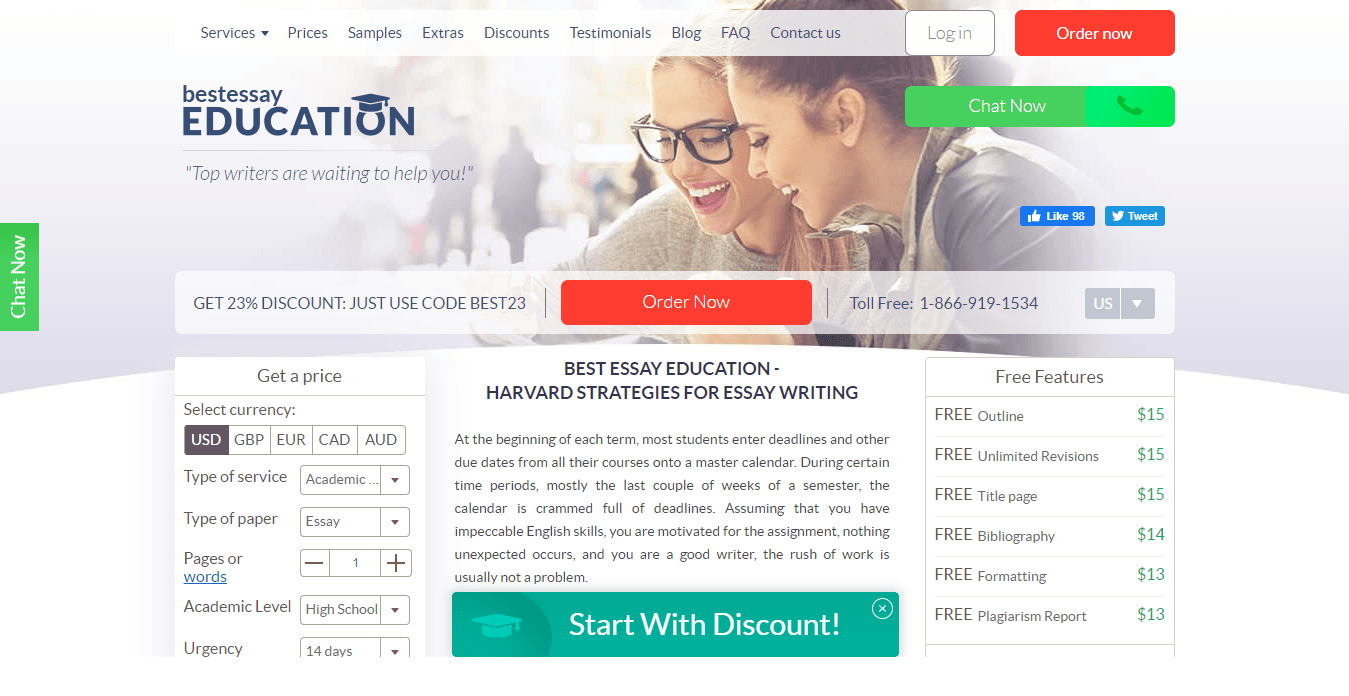**Image Caption:**

Top Plus offers a wide range of academic services, featuring competitive prices, sample extras, and exclusive discounts. Numerous testimonials endorse their offerings. A distinctive red rectangle prompts viewers to "Order Now," while another declares "Best Essay Education" with top writers ready to assist.

In the background, students are engaged in a lively discussion, smiling as they collaborate. A blue rectangle nearby encourages viewers to "Like" with a counter showing 98 likes and a "Tweet" option. There's an enticing offer of a 23% discount with the use of code BEST23.

Additionally, a toll-free number (1-866-919-1534) is highlighted for convenience. The service options include selecting currency types such as USC, GPP, EOR, CAD, and EOD. The academic service includes writing essays at the high school level with options for pages or words specified, with an origin deadline of 14 days. Complimentary offerings include final revision, title page, bibliography, and formatting.

The pricing is detailed, with specific costs of $15, $50, $40, and $30 listed. Toward the end of each term, students typically mark their deadlines on a master calendar, which becomes particularly congested in the final weeks. Assuming strong English skills and motivation, meeting these requirements should not be an issue for a good writer. Another green rectangle emphasizes starting with a discount.